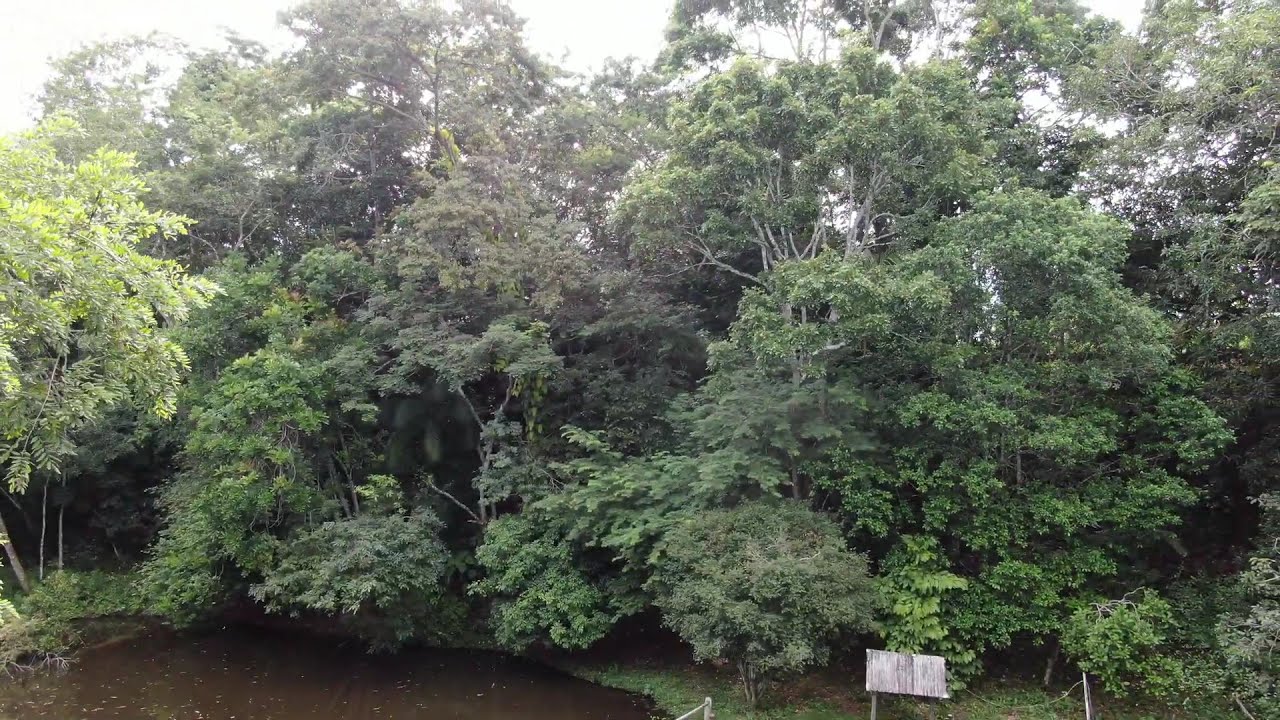This aerial photograph, taken during a partly cloudy day, reveals a lush, densely vegetated area dominated by numerous tall trees in full leaf, showcasing various shades of green and hints of yellow from possible flowers. The sky, though partly visible, appears predominantly white due to the cloud cover. Situated on the left side of this rectangular image is a murky pond with dark brown water, its surface speckled with floating leaves. The bottom part of the photograph includes a roped-off area and a worn wooden sign, suggesting that this could be part of a zoo, sanctuary, or perhaps a hiking park. The backdrop is a thick, almost impenetrable forest that adds to the outdoor aesthetic of the scene.